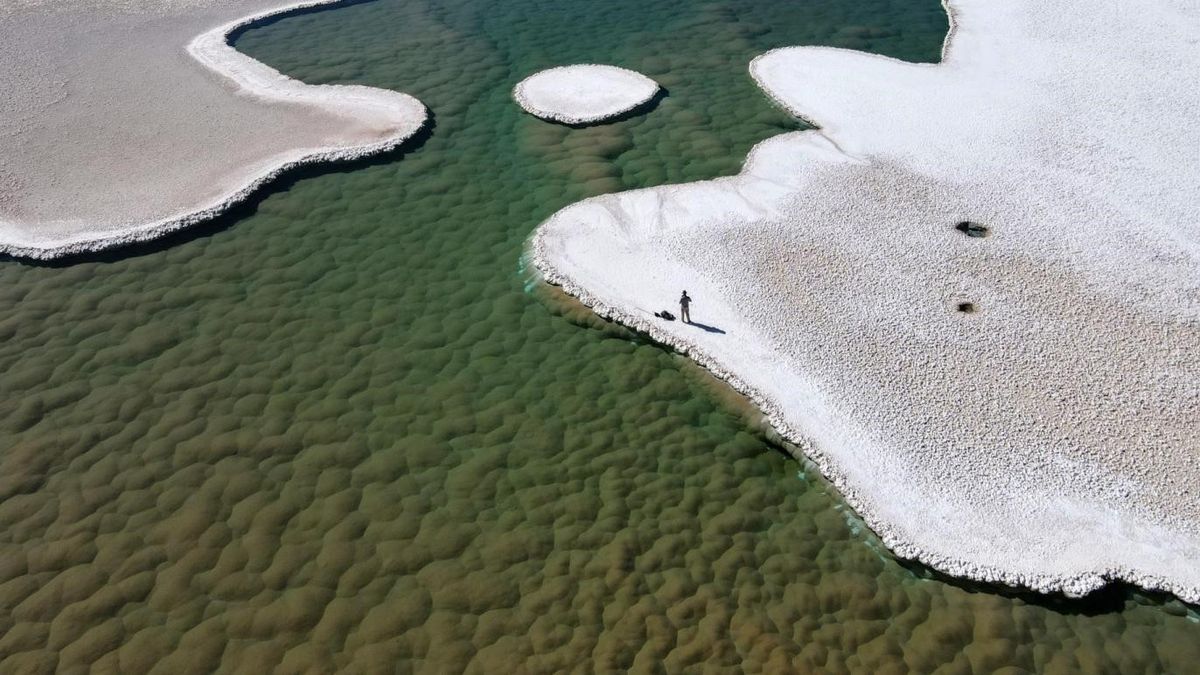Aerially shot from a few hundred feet, this intriguing image captures a person standing on what seems to be white salt or lime deposits forming curvy, flat formations along the edges of a green, bumpy, watery terrain. These white formations, strikingly bright on the edges and darker towards the center, hug the outermost parts of the image. Central to the scene is a small circular white island, further accentuating the unique landscape. The water, a dark and murky green, appears densely covered with moss or algae, adding to the abstract texture. The lone figure's shadow extends to the right, with something small lying on the ground beside them, perplexing and enhancing the enigmatic nature of the photograph.